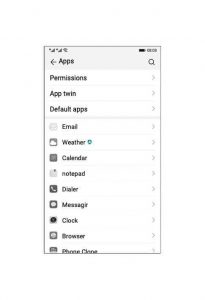Detailed Caption: 

The image depicts a screenshot of a settings interface, presumably from a device. The background of the screen is plain white. At the very top, the main header reads "Apps" positioned in the left corner along with a right-pointing arrow. On the right side of this header is a search box, identifiable by the small magnifying glass icon on its edge.

Beneath the header, a series of drop-down menus related to app settings are listed. The first menu labeled "Permissions" is on the left, with a clickable drop-down arrow on the right. Following this is the "App Twin" menu, similarly formatted with a drop-down option. Below that is another drop-down menu for "Default Apps."

Dividing these sections is a horizontal gray line serving as a border. Under this border, the lower section of the interface lists several app categories, each accompanied by a recognizable icon. The apps displayed include "Email," "Weather," "Calendar," "Notebook," "Dialer," "Messenger," "Clock," "Browser," and a partially visible option starting with "Phone."

Each icon next to the app names is monochromatic, except for the "Weather" icon, which includes a small green dot, adding the only splash of color to the otherwise black and white interface. The details are somewhat blurry, especially the section labeled "Phone something," but the image remains decipherable overall.